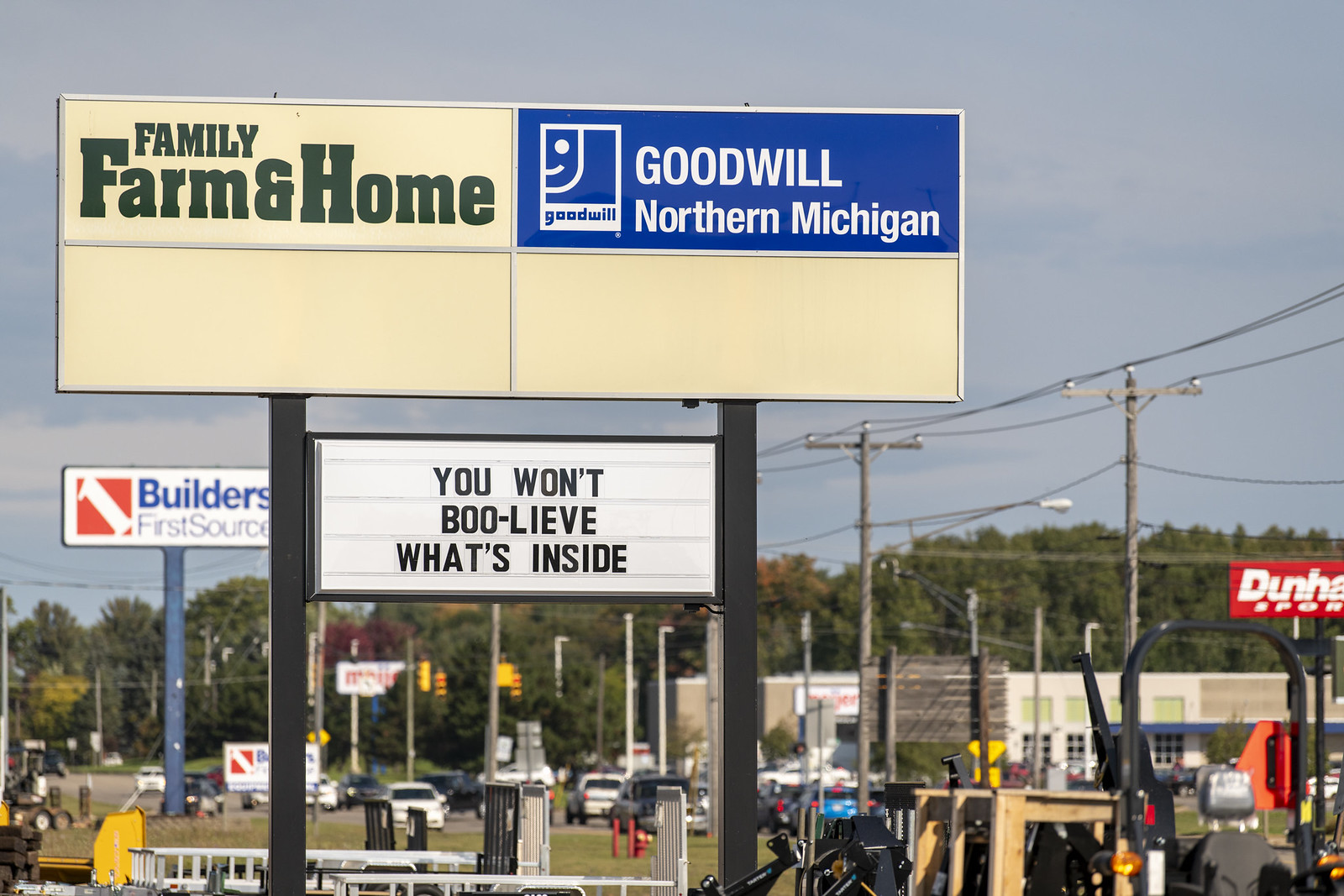In the bustling shopping district, a prominent sign stands in the foreground, featuring "Family Farm and Home" at the top. Adjacent to it, a smaller square sign for "Goodwill Northern Michigan" humorously displays, "You won't boo-lieve what's inside," hinting at a Halloween-themed promotion. To the right, another sign for "Builders First Source" is visible. The foreground is dotted with tractors and various lawn equipment. Across the street, the background reveals a variety of indistinct businesses. Traffic lights and a few cars punctuate the scene, highlighting the busy street that separates the onlooker from the commercial establishments.